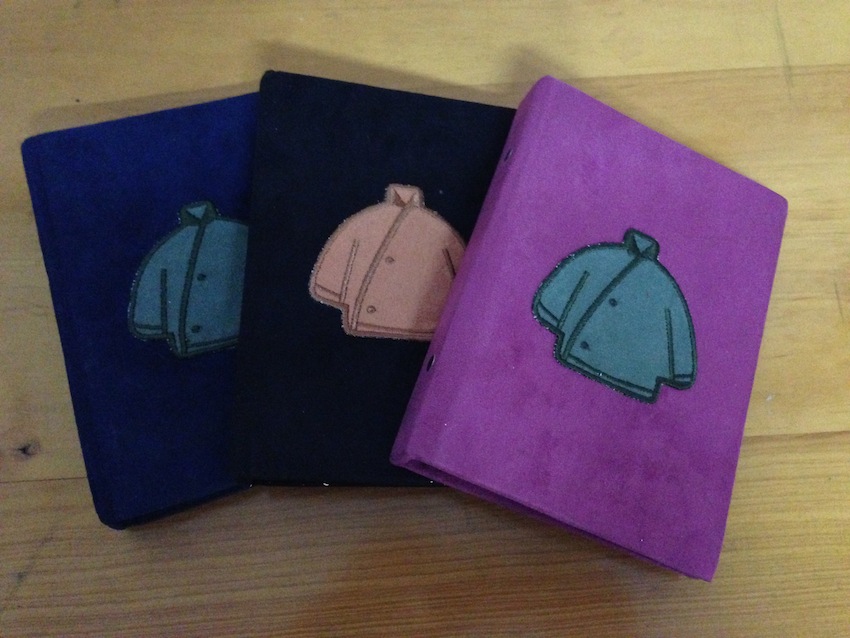The photograph captures three cloth-bound journals laid out on a blond wood table, taken from a top-down perspective. Each journal features a cover with a texture resembling either microsuede or velour, providing a soft, fabric-like appearance. The journals are slightly stacked at an angle, allowing all of them to be fully visible. Each journal is distinct in color and has an embroidered or sewn patch on its cover, depicting a collarless chef's-type jacket that wraps over rather than buttoning down the middle and features two buttons. 

The journal on the left is dark blue with a light blue jacket applique, the middle journal is black with a beige jacket applique, and the rightmost journal is a rich violet-purple with another light blue jacket applique. The detailed contrast of colors and textures against the wooden surface highlights the intricate design and craftsmanship of these unique book covers.